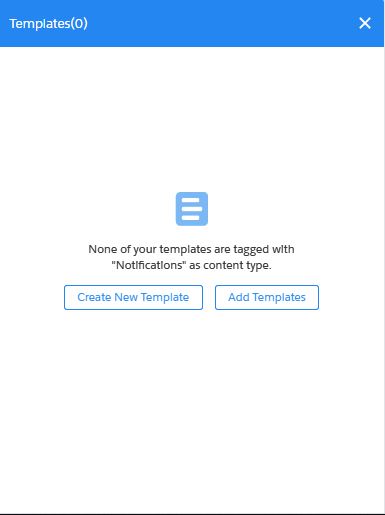In the upper left corner of the digital image, the word "Templates" is displayed in a white font. Adjacent to it, enclosed in parentheses, is the number "0". At the top of the image, a solid blue bar stretches across, measuring approximately one inch in height and several inches in length. In the top right corner of this blue bar is a small white "X".

Centrally positioned within the main body of the image, there's a notification that reads, "None of your templates are tagged with 'Notifications' as content type." Below this message, two buttons are visible. The first button, labeled "Create New Template," is positioned to the left, while the second button, labeled "Add Templates," is situated to the right of the first button.

At the bottom of the image, there is a long, straight black line that spans across the width.